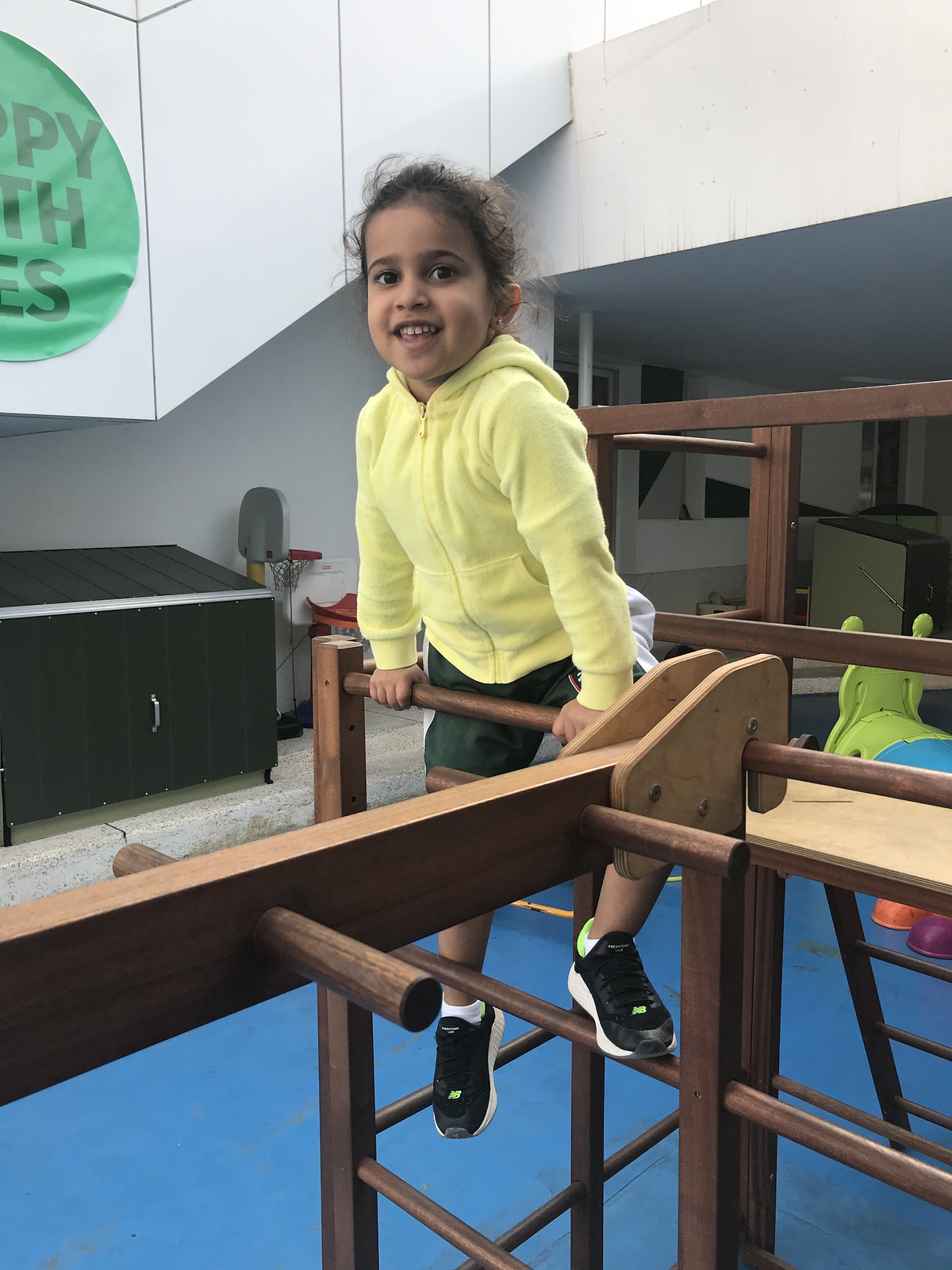The image captures a lively scene of a young girl, aged approximately four to six years old, energetically climbing an indoor wooden jungle gym. She stands confidently on the monkey bar-like ladder, posing with a joyful expression for the camera. Dressed in green shorts, a yellow sweatshirt, and sneakers, the girl has dark hair, brown eyes, and an olive complexion. The room around her features plain white walls and a variety of children's play equipment, including more wooden playground structures and a frog-shaped ride-on toy. A vivid detail is the blue safety mat on the floor, designed to cushion any falls. In the back, there is a closed storage bin and some sports equipment lining the walls. Noteworthy is a partially visible circular banner with black lettering and a green half-circle sign with text that is cut off, adding a sense of mystery to the setting. The upper part of the image also hints at a staircase or an incline, emphasizing the multi-level nature of the space.